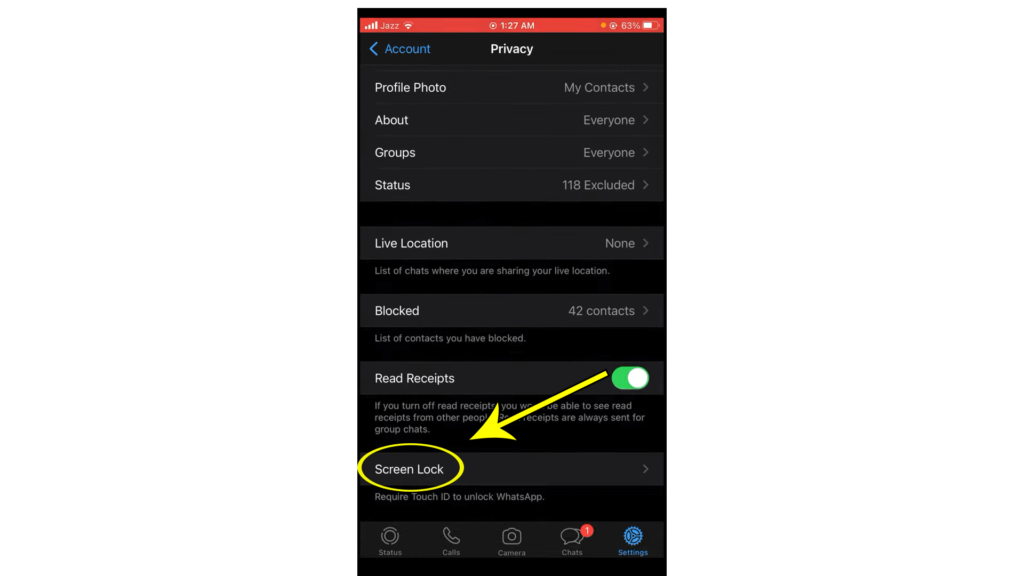The image displays a smartphone interface focusing on the settings page with a dark theme background. 

In the top bar, on the left side, there is a red indicator bar and the reception status showing "Jazz" alongside a Wi-Fi symbol. The time is displayed as "1:27 a.m." On the right side, it shows the battery level at 63%.

Below, in the settings menu, the section headers and items are presented in a structured format. 

- The "Account" heading is highlighted in blue at the upper left. Below that:
  - "Privacy" is the main heading in bold, leading into a detailed list of privacy settings.
  - "Profile Photo" with "My Contacts" on the right.
  - "About" with "Everyone" on the right.
  - "Groups" with "Everyone" on the right.
  - "Status" with "118 Excluded" on the right.

Further down:
- A section titled "Live Location" indicating "None," followed by a description that reads "List of chats where you are sharing your live location."
- "Blocked," showing "42 contacts," and a note saying "List of contacts you have blocked."

In another section:
- The "Read Receipts" setting is shown in white with a green toggle button turned on. A yellow arrow points from this button to the next section.

- "Screen lock" features a yellow circle around it, indicating the option "Require Touch ID to unlock WhatsApp."

At the bottom of the screen, there is a navigation bar with icons labeled as "Status," "Calls," "Camera," "Chats," and "Settings."